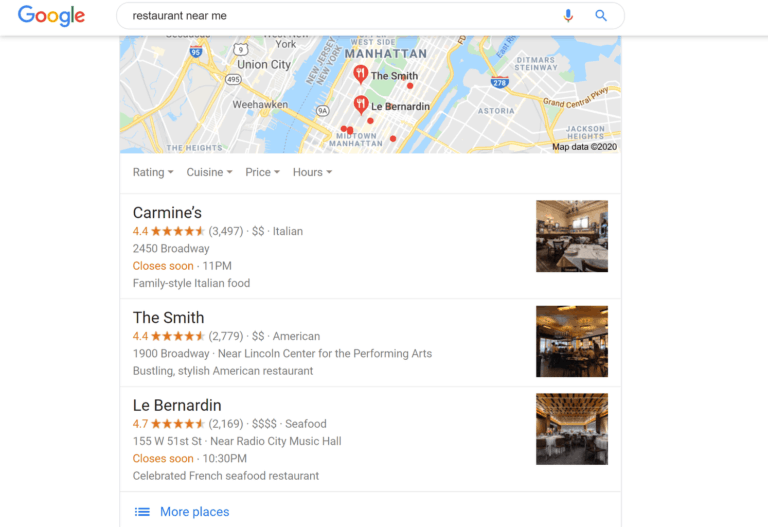The image depicts a Google search page, where the term "restaurant near me" has been entered, specifically focusing on the Manhattan area. The search results showcase three restaurants: Carmine's, The Smith, and La Bernarda. Each listing includes a star rating, the restaurant's address, the type of cuisine offered, and a brief description. Additionally, to the right of each listing, there is a photo displaying the interior of the respective restaurant, inviting viewers to get a sense of the ambiance and decor.